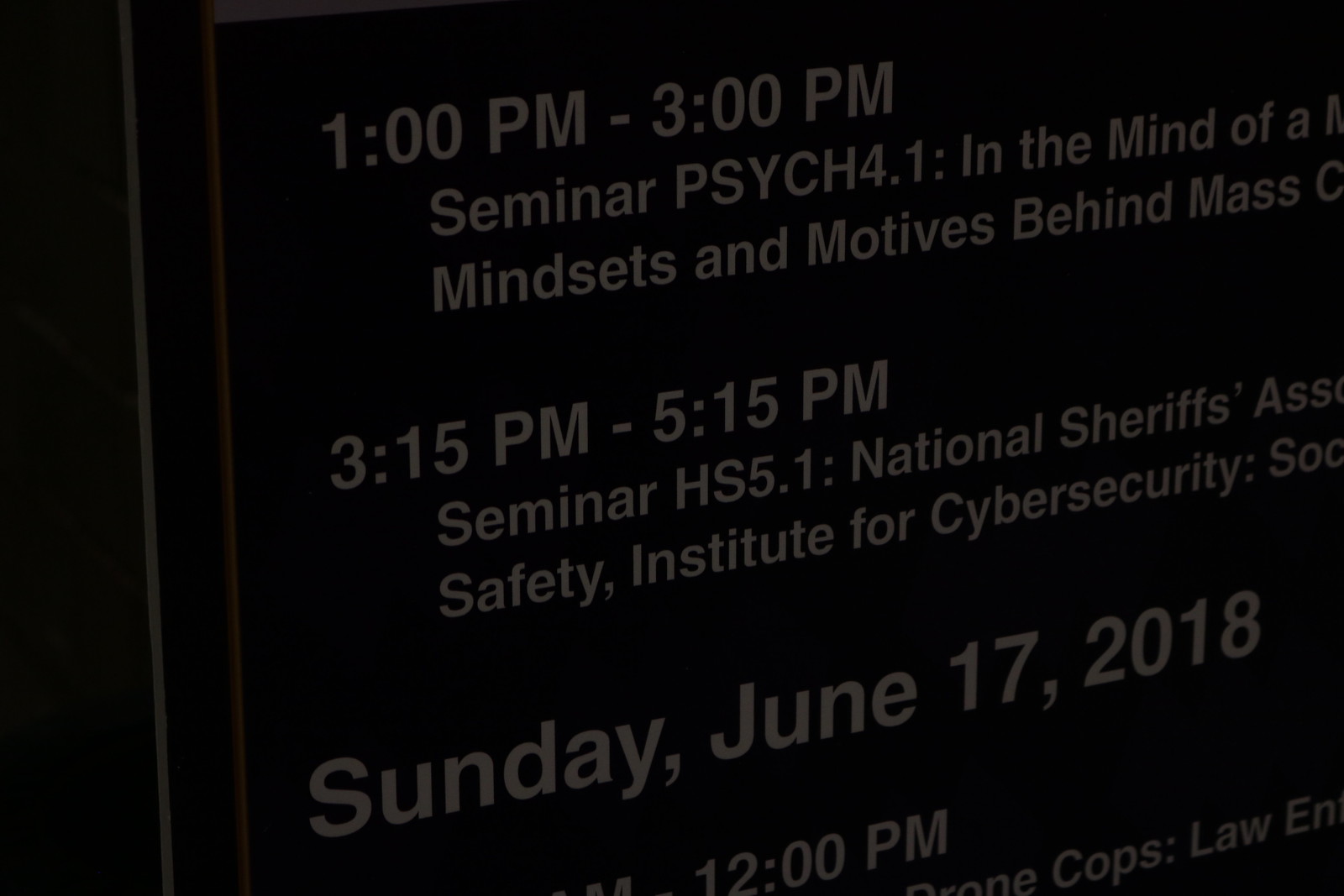The image displays a detailed schedule on a digital screen with grey text on a black background, possibly from an expo or convention. The schedule starts with a seminar from 1 p.m. to 3 p.m. listed as "Psych 4.1: In the Mind of," which is partially cut off, followed by a session titled "Mindsets and Motives Behind Mass," also incomplete. The next entry from 3:15 p.m. to 5:15 p.m. is another seminar labeled "HS 5.1: National Sheriff's," truncated, likely indicating "Association," followed by "Safety Institute for Cybersecurity," with the rest of the text cut off. The schedule proceeds to Sunday, June 17th, 2018, showing an event at 12 p.m., partially mentioning "drone cops law," cut off at the end. The screen has a gray border framing the schedule, enhancing the contrast against the dark background.